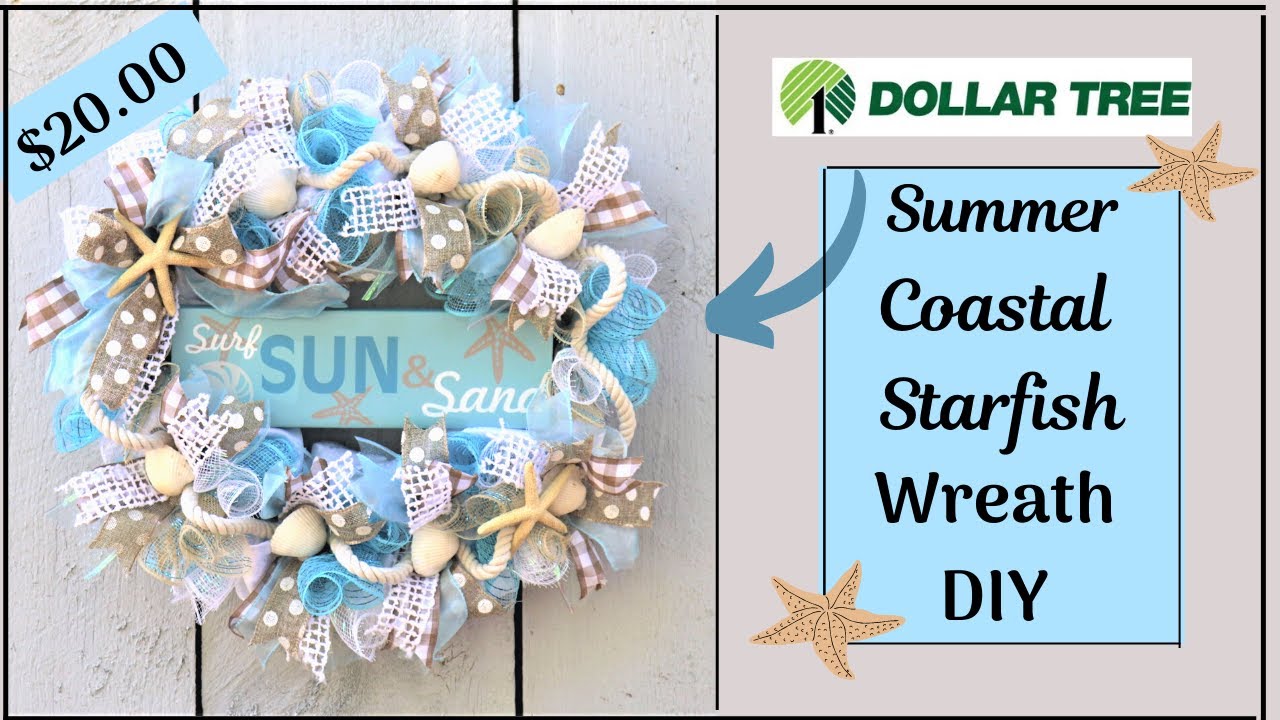This advertisement for Dollar Tree features a beautifully crafted Summer Coastal Starfish Wreath DIY, showcased against a backdrop designed to resemble a white plankboard wall for a nautical feel. Prominently placed in the top right corner is the recognizable Dollar Tree logo with its green tree icon and distinct font. Below the logo, a blue rectangle reads "Summer Coastal Starfish Wreath DIY" with two pink starfish in the corners and an arrow pointing to the left, directing attention to the wreath. The wreath itself, priced at $20 as noted in a blue banner at the top left corner of the image, is an exquisite assembly of light blues, whites, and tans. It features starfish and various ribbons—including natural-toned, polka-dot, airy canvas, and gingham patterns—interwoven with light-colored rope and transparent blue ribbon. A central wooden sign in light blue, adorned with more starfish, proclaims "Surf, Sun, and Sand," completing the charming coastal theme.